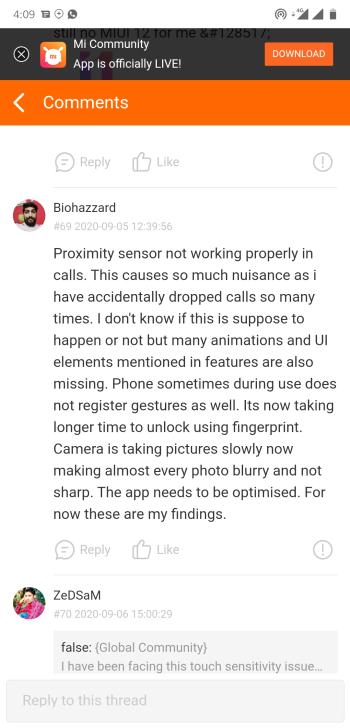This image showcases a screenshot of the "Mi Community" app interface. At the top of the screen, the title "Mi Community" is prominently displayed, indicating the app is officially live. To the right of the title, there is an orange download button. On the left side of the title, there is an "X" button. Just below the title, an orange bar featuring the word "Comments" in white text is visible, alongside a back button.

Beneath the header, there's a comment section with a white background. The first comment is from a user named "Biohazard," whose profile picture is displayed to the left of their comment. Biohazard details various issues they have encountered, including a malfunctioning proximity sensor during calls, accidental call drops, missing animations and UI elements, unregistered gestures, delayed fingerprint unlocking, and camera performance issues resulting in blurry photos. Biohazard concludes by stating that the app needs optimization and lists these findings.

Following Biohazard's comment, another user has replied, indicating that Biohazard's issues are false.